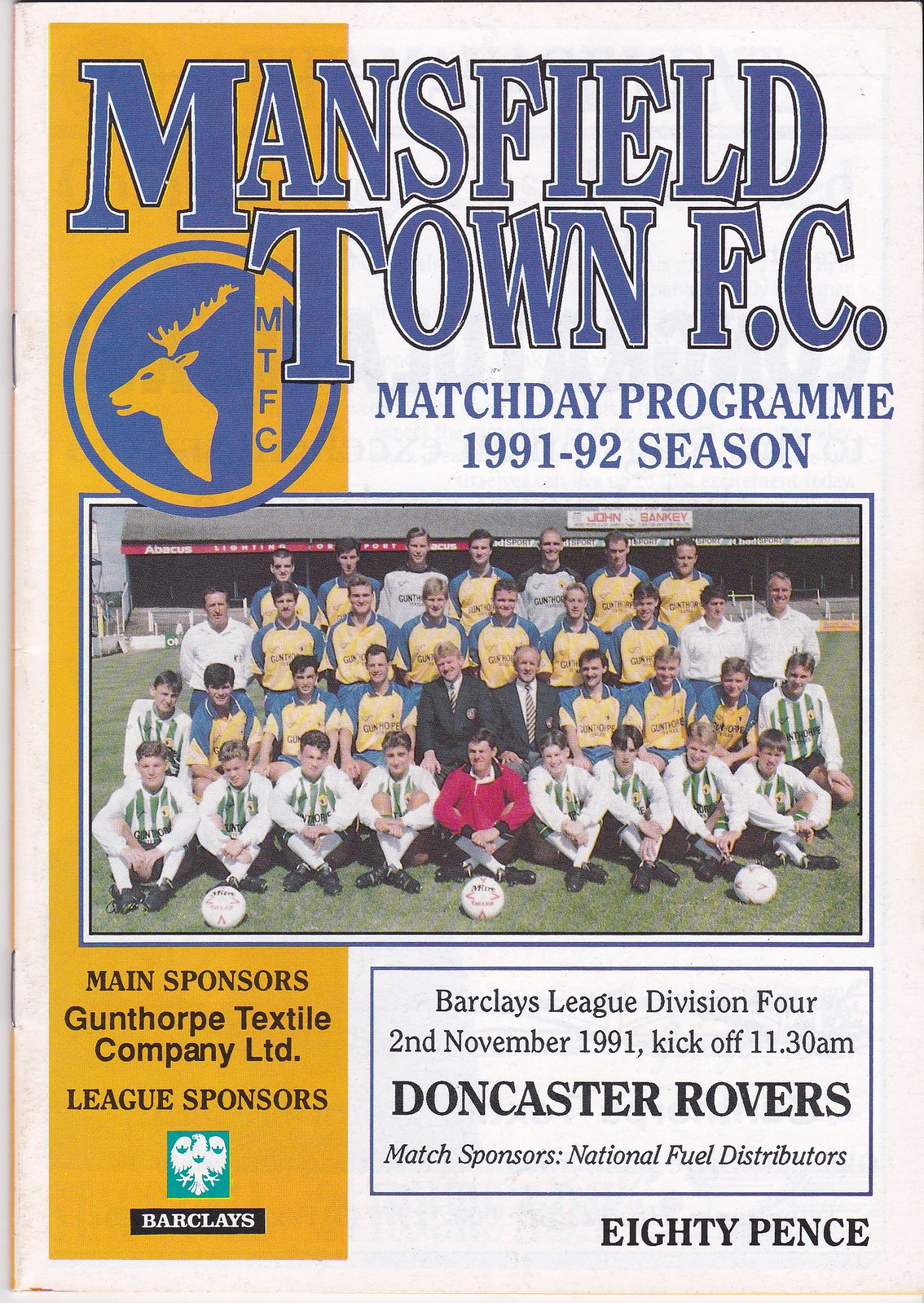This image features the cover of a vintage Match Day Program from the 1991-92 season for Mansfield Town FC. The top prominently displays "Mansfield Town FC" with a blue circular logo featuring a yellow deer head and "MTFC" text. A yellow vertical strip runs down the left side. The center showcases a team photograph with players in yellow and blue jerseys, arranged in four rows – the back rows standing and the front rows seated. Two men in suits, likely the coaches, are positioned among the team, with goalkeepers and officials also present. The setting appears to be on a football field. Notable details include the headlines "Match Day Program 1991-92 season," main sponsors "Gunthorpe Textile Company Limited," league sponsors "Barclays League Division IV," and information about the match: "2nd November 1991, kickoff at 11:30 AM," against Doncaster Rovers, with match sponsors "National Fuel Distributors." The price is marked as "80 pence."